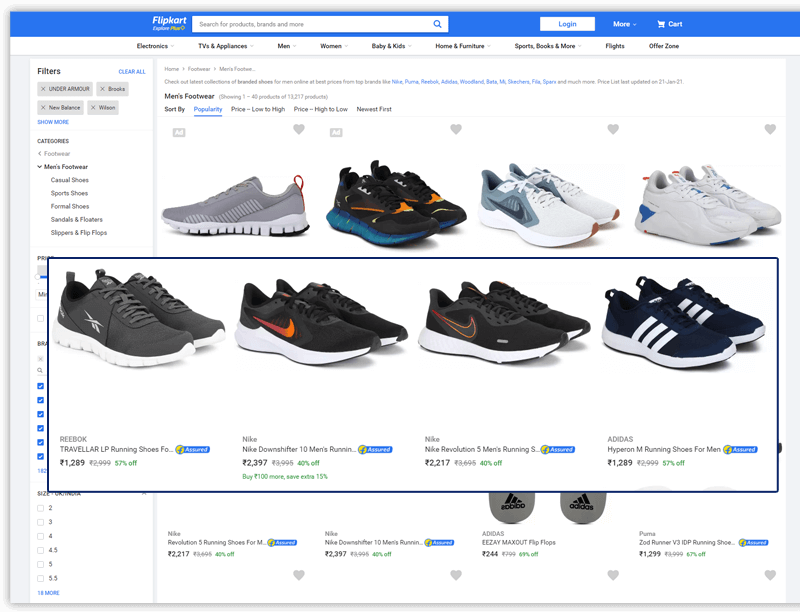This image is a screenshot from the online shopping platform Flipkart, featuring a page dedicated to tennis shoes. The page is titled "Flipkart Express, Flipkart Explore Plus," with the brand name clearly spelled out as "Flipkart" (F-L-I-P-K-A-R-T). At the top of the page, there is a search bar labeled "Search for products, brands and more," allowing users to easily find items. Next to the search bar, there are buttons for "Login" and "More" with a drop-down menu, as well as a shopping cart icon accompanied by the text "Cart."

Below the top navigation bar, the site categorizes products into sections like "Electronics," "TV and Appliances," "Men," "Women," "Baby and Kids," "Home and Furniture," "Sports, Books, and More," alongside special sections for "Flights" and "Offer Zone."

The main focus of the page is a display of tennis shoes with two rows of products. Each row features four pairs of shoes. The second row appears to be highlighted, perhaps indicating that a user has clicked on it. This row is enclosed by a thick, deep navy blue to black rectangle.

The highlighted shoes include:
1. Reeboks Traveler LP running shoes,
2. Nike Downshifter 10 men's running shoes,
3. Another model of Nike shoes,
4. Adidas running shoes.

The detailed presentation of the products and navigation options highlights the comprehensive shopping experience offered by Flipkart.